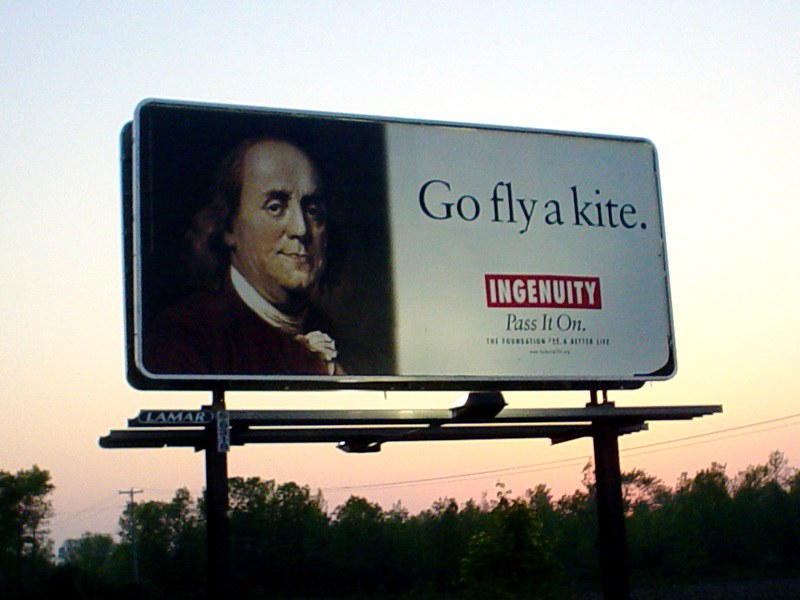The billboard features a prominent image of Benjamin Franklin against a dark background on the left side. To the right, a white background showcases the phrase "Go fly a kite" in bold lettering. Below this, a red rectangular box contains the word "Ingenuity" in white text, followed by the phrase "Pass it on" in smaller font beneath. At the lower part of the billboard, dark green trees are visible, their lush foliage creating a natural contrast. Supporting the sign is a black-framed base with horizontal dark gray beams, marked with "Lamar" in white on the left side. The backdrop of the image blends from a subtle pink hue at the bottom of the sky, transitioning smoothly into a lighter white shade towards the top.